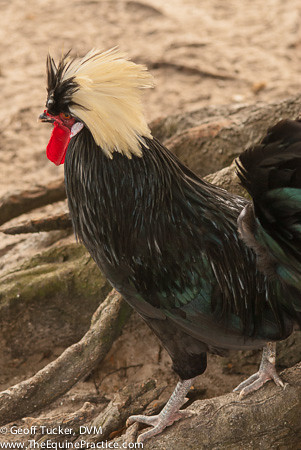This detailed image, captured by Geoff Tucker DVM and available at www.theequinepractice.com, features a striking rooster perched on a rock formation adorned with green moss. The rooster boasts a commanding presence with its white feathery head contrasted against a black face and a pronounced red wattle. Its impressive plumage includes long feathers in shades of black, teal, and emerald green. The rooster's large tail feathers mirror the vibrant hues of its body. It stands on white-clawed feet, set against a background of earthy tree roots and dirt, suggesting a natural, wild setting. The composition is completed with a copyright notice in the bottom left corner, in white text.